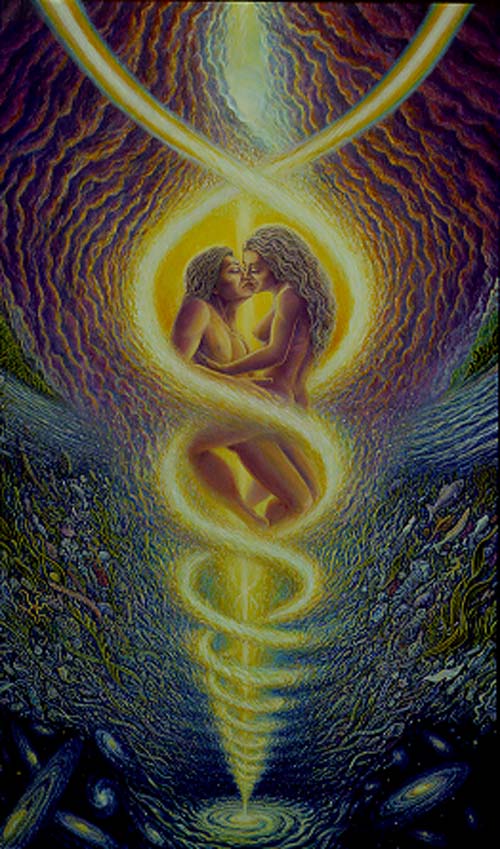This vertical painting features two naked women with long, blondish hair and darker skin, passionately embracing and kissing amid an abstract, vibrant scene. The women appear suspended or rising, potentially from water or in a cosmic void, highlighted by swirling, golden lines reminiscent of a twisting medical symbol. Surrounding them are diverse, multicolored backgrounds with purples, blacks, and greens, interspersed with galaxies and stars. The artwork, filled with intricate designs and shapes, bears resemblance to Alex Gray's style, blending vivid, wave-like colors and potentially aquatic elements such as fish and leaves.